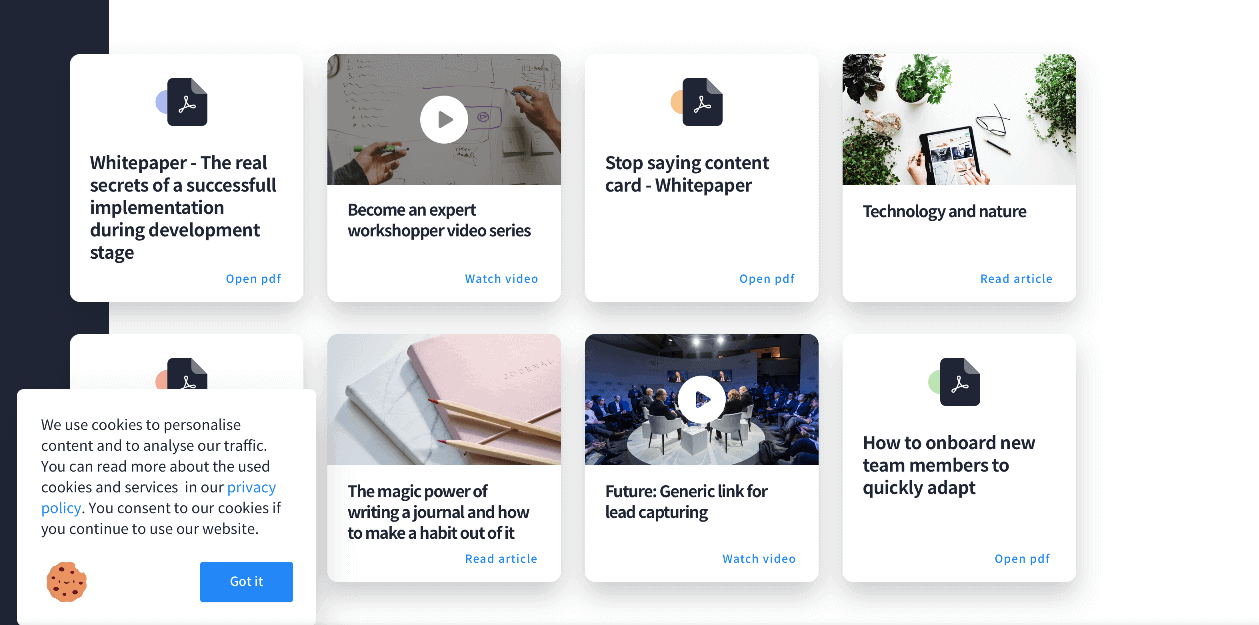The image depicts a section of an Adobe website, specifically an informational or tutorial section. The layout is organized into eight square tiles, with four tiles positioned at the top row and four at the bottom row. A distinguishing feature is a vertical black bar approximately 1.5 inches wide, running along the left side of the image.

Each white tile contains distinct content:

1. The top left tile features a black sheet with the Adobe logo in white, titled "The Real Secrets of Successful Implementation During Developmental Stages."
2. The next tile displays an instructional video labeled "Watch to Become an Expert Workshopper."
3. The following tile is titled "Stop Saying Content Card."
4. The fourth tile reads "Technology and Nature."

On the bottom row:

1. The bottom left tile is partially obscured by a cookies consent pop-up.
2. The next tile is about "The Magic Power of Writing a Journal and How to Make a Habit Out of It."
3. Following this, one tile is a placeholder labeled "Future Generic Link for Lead Capturing."
4. The final tile provides information on "How to Onboard New Team Members to Quickly Adapt."

Overall, the image displays a structured, user-friendly interface designed to guide users through various topics and resources related to Adobe.